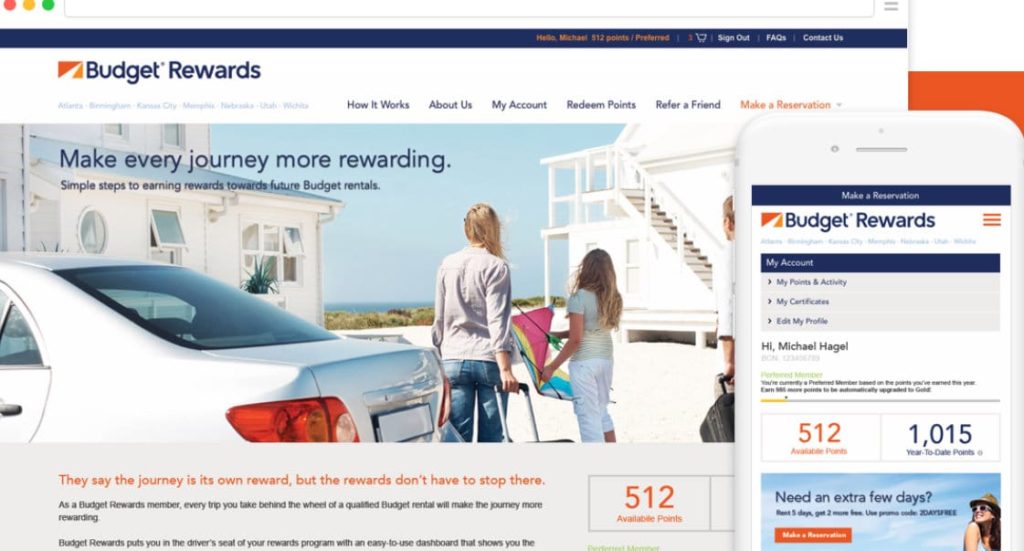This image is designed for the "Budget Rewards" website, featuring the company logo prominently in the top-left corner. The logo consists of an orange rectangle split diagonally: the upper quadrant is dark orange, while the lower quadrant is light orange, with a white stripe cutting through it. To the right of the logo, the company's name "Budget Rewards" is boldly displayed in large, dark blue text.

Central to the website is a large, captivating image depicting a picturesque vacation scene. In the foreground, there is a family of three—a woman, a man, and a young girl—standing beside their vehicle. On each side of them, pristine white beach houses are visible, indicating a serene and idyllic vacation spot. The beach itself, along with a beautiful blue skyline, stretches out in the background, adding to the overall sense of relaxation and adventure.

Overlaying the top-left of the image is a piece of text that reads, "Make every journey more rewarding. Simple steps to earn rewards towards future Budget rentals." This tagline emphasizes the benefits of using the service for future vacation plans.

Additionally, to the right side of the website, there is an image of a smartphone displaying the Budget Rewards app interface. At the bottom of the smartphone screen, an icon with the text "Need an extra few days?" suggests extended rental options for users, further catering to travelers' needs.

Overall, the image encapsulates the essence of Budget Rewards—a convenient service tailored for families eager to make their vacation experiences more rewarding through simple, beneficial steps.